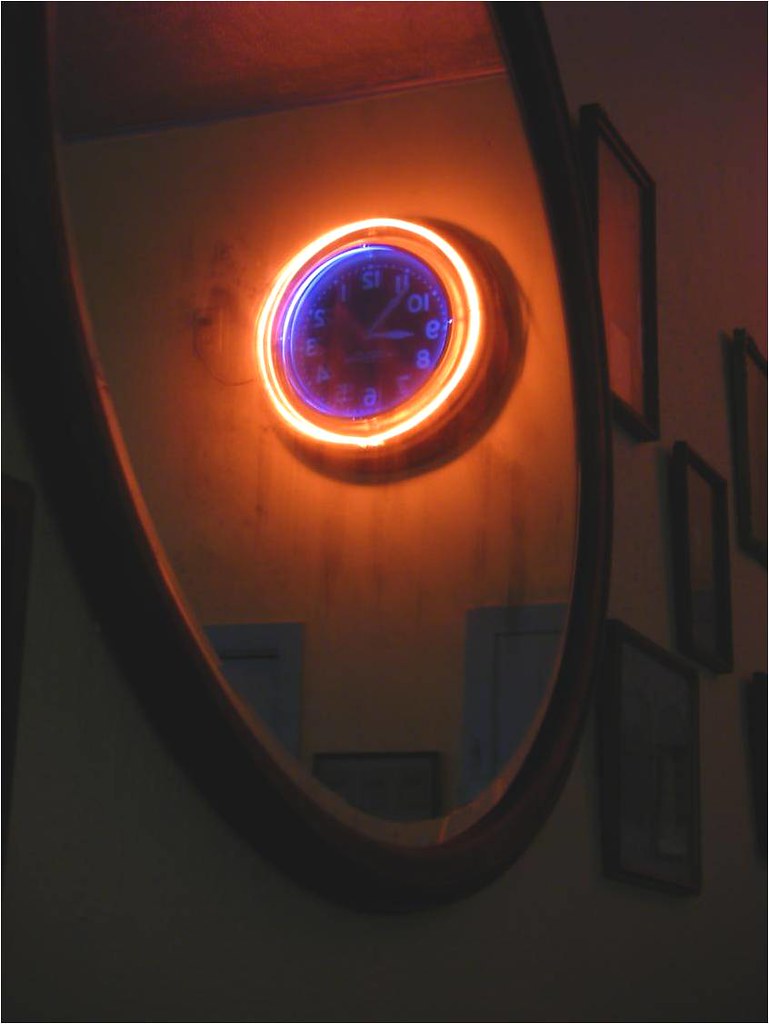In this photo taken inside a dimly lit home, a round or oval mirror mounted on a white wall captures a reflection of a vintage-style clock. The scene appears to be a close-up shot with the lights off, but there is enough ambient light to discern details. The clock, centrally positioned in the mirror's reflection, is illuminated, resembling a neon glow with multiple concentric circles of light. The innermost circle glows yellow, followed by a surrounding circle of orange light. The clock hands stand out against a black background, contrasting starkly with the illuminated colors. Above the clock, five or six small to medium-sized picture frames are closely arranged, although their specific contents are indistinct. The overall ambiance of the image is one of cozy intimacy, emphasizing the details of the clock and the decorative arrangement on the wall.